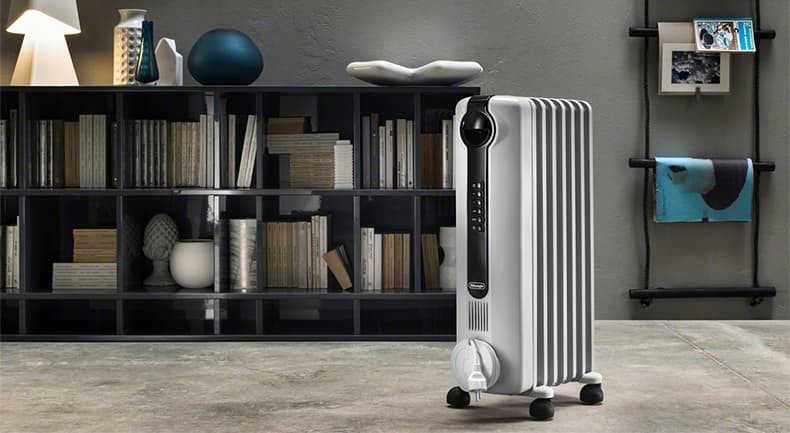The photograph, taken indoors in landscape mode, features a sleek, rectangular appliance with curved edges, standing approximately 2 to 3 feet high on short wheeled legs. This white or silver device, possibly an air purifier or air conditioner, has a black stripe down the middle that likely contains control buttons, and a small vent and plug near the bottom. In the foreground, you can see its smooth, modern design. The background reveals a room with a stone floor and gray walls. Prominently on the right side is a ladder-style décor piece, draped with art and a brochure. To its left stands a black bookcase with 8 to 10 cubbies filled mostly with books displayed spine out, along with some decorative items. Atop the bookcase are various sculptures including a white reclining figure, a blue orb, a white and blue vase, and a white lamp, adding to the room’s contemporary style.